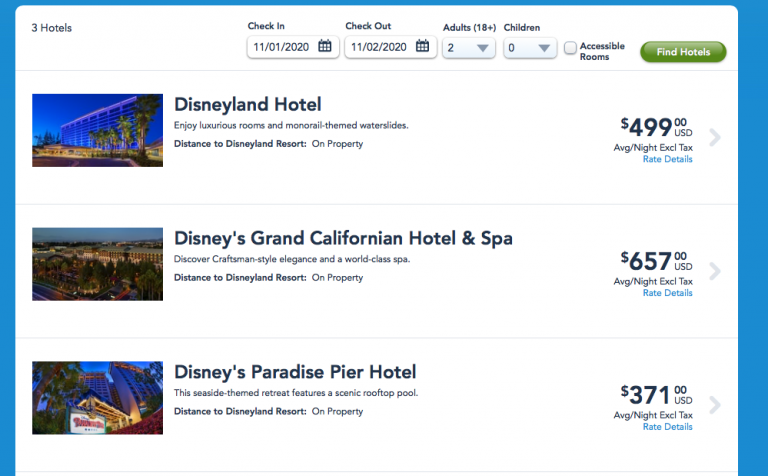The image displays promotional content for three Disney hotels against a blue background with a white central section. In the upper left corner, there is a header with "Three Hotels" written within a small blue-bordered box. Below this, details for a sample booking can be seen: "Check-in: 11/01/2020", "Check-out: 11/02/2020", "Adults: 2", "Children: 0", "Accessible rooms: Unchecked," followed by a green button labeled "Find Hotels."

The main portion beneath this booking information showcases three distinct Disney hotels with detailed descriptions and images:

1. **Disneyland Hotel**:
   - Description: Enjoy luxurious rooms and monorail-themed water slides.
   - Distance to Disneyland Resort: On property.
   - Price: $499 per night.

2. **Disney's Grand Californian Hotel and Spa**:
   - Description: Discover craftsman-style elegance and a world-class spa.
   - Distance to Disneyland Resort: On property.
   - Price: $657 per night.

3. **Disney's Paradise Pier Hotel**:
   - Description: This seaside-themed retreat features a scenic rooftop pool.
   - Distance to Disneyland Resort: On property.
   - Price: $371 per night.